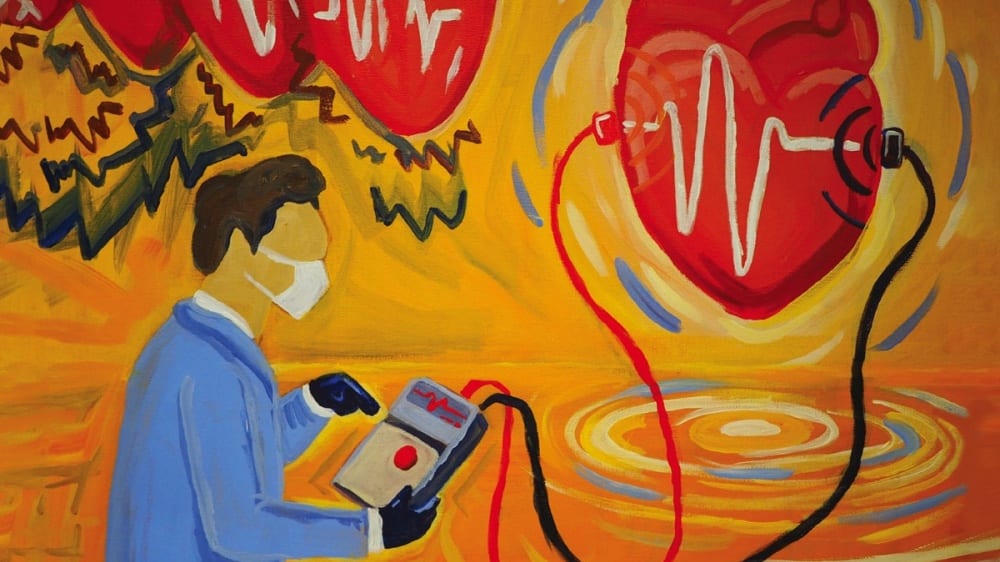The painting depicts a doctor on the left side, dressed in a blue suit and wearing a white face mask. The doctor is holding a heart monitor device in his right hand, characterized by a single red button and two wires—red on the left and black on the right—that connect to a large red heart on the top right of the painting. The device and the heart both feature an ECG (electrocardiogram) line. The heart appears to be over a water-like surface, causing a ripple effect beneath it. The background is a bright orange hue, which contrasts with the vivid blue suit of the doctor. Above the doctor, on the left side, there are graffiti-like jagged blue and brown lines, alongside overlapping hearts drawn similarly to the prominent large heart. This collection of elements suggests a medical theme interwoven with an artistic representation of heart activity and vitality.